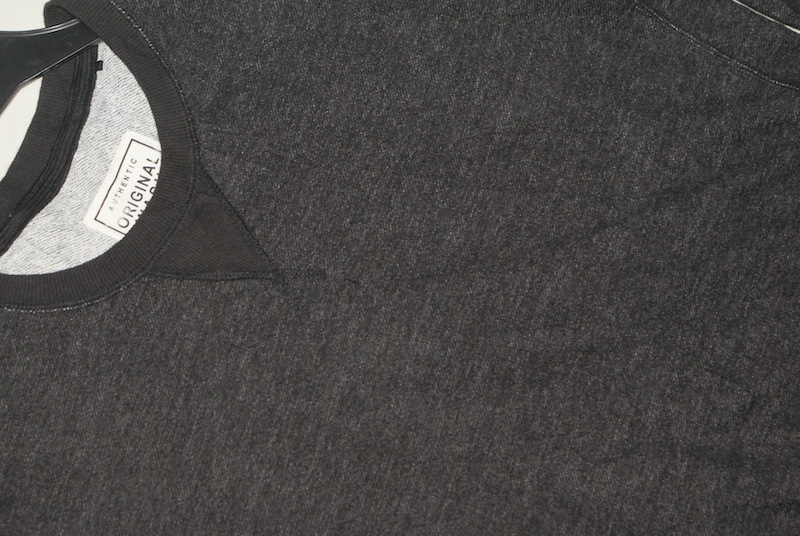The photograph, meticulously cropped to focus on the upper portion of the garment, depicts a dark heathered gray shirt displayed on a black plastic hanger. Centered in the frame is the shirt's crew neck collar, which is a solid dark gray and features a distinctive triangular reinforcement at its base, with the broad side of the triangle hugging the collar's edge and the pointed tip directed downward. The inner fabric, visible around the collar's rim, is a light heather gray, adding a faint contrast to the main body of the shirt. Adorned on this inner fabric at the back is a white tag outlined in black, which bears the partial phrase "authentic original" in black lettering. The crop of the image excludes the sleeves, sides, and hem of the shirt, drawing the viewer's attention to the intricate details of the upper garment construction.